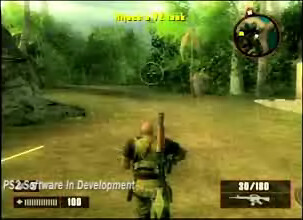The image is a color screenshot from a military-themed computer game, showcasing a scene with noticeable blurriness and pixelation. At the center of the image, we see the back of a soldier dressed in camouflage gear. A large, cylindrical weapon is securely fastened vertically to his back. The soldier is positioned on a wide, brown path that resembles either a dirt road or a dried-up riverbed, which curves to the left towards the middle of the screen. Blurry green trees line both sides of this path, adding to the natural environment. In the bottom left-hand corner of the image, white text reads "PS2 software in development," indicating that this might be an early or unfinished version of the game. In the lower right-hand corner, there is a dark rectangle displaying the numbers "30-180" alongside a silhouette of a rifle, suggesting in-game information, possibly related to ammunition or an objective marker.